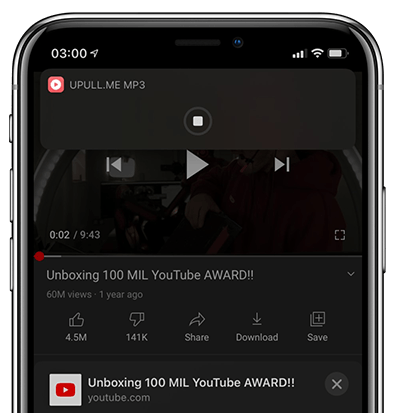This image depicts the detailed top view of a sleek, black, shiny cell phone. The phone has three buttons on the left side, likely for volume control and other functions, and a single button on the right side. On the screen, we can see the time displayed in the top left corner, reading "03:00," accompanied by a paper airplane icon. Moving across the top of the screen, signal strength bars, a Wi-Fi icon, and a partially filled battery indicator, which appears around 80-90% full, are visible.

Beneath these status icons, the screen shows a YouTube video titled "Unboxing 100 MIL YouTube Award," which is currently paused at two seconds into its nine-minute and 43-second duration.